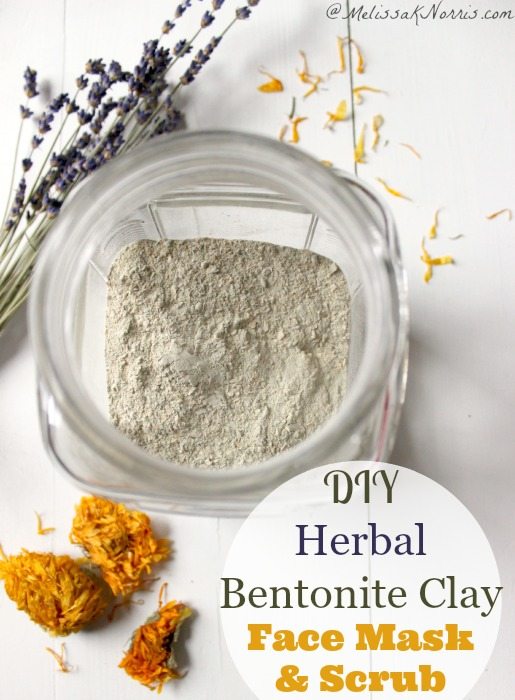The image showcases a do-it-yourself herbal bentonite clay face mask and scrub. The setup features a transparent glass jar in the center, containing a powder, presumably the bentonite clay. The text "DIY Herbal Bentonite Clay Face Mask and Scrub" is prominently displayed in a circle, with the word "DIY" in green, "herbal bentonite clay" in black, and "face mask and scrub" in yellow. The jar sits on a white plank countertop. Surrounding it are sprigs of lavender with light green stems and tiny purple flowers, broken yellow leaves, and dried yellow-orange flowers. Above the jar, towards the left, more lavender and yellow-orange petals are visible. At the top of the image, the text "at Melissa Norris dot com" indicates the creator of the content, suggesting that the powder and accompanying herbs are components of the homemade face mask featured on her website.